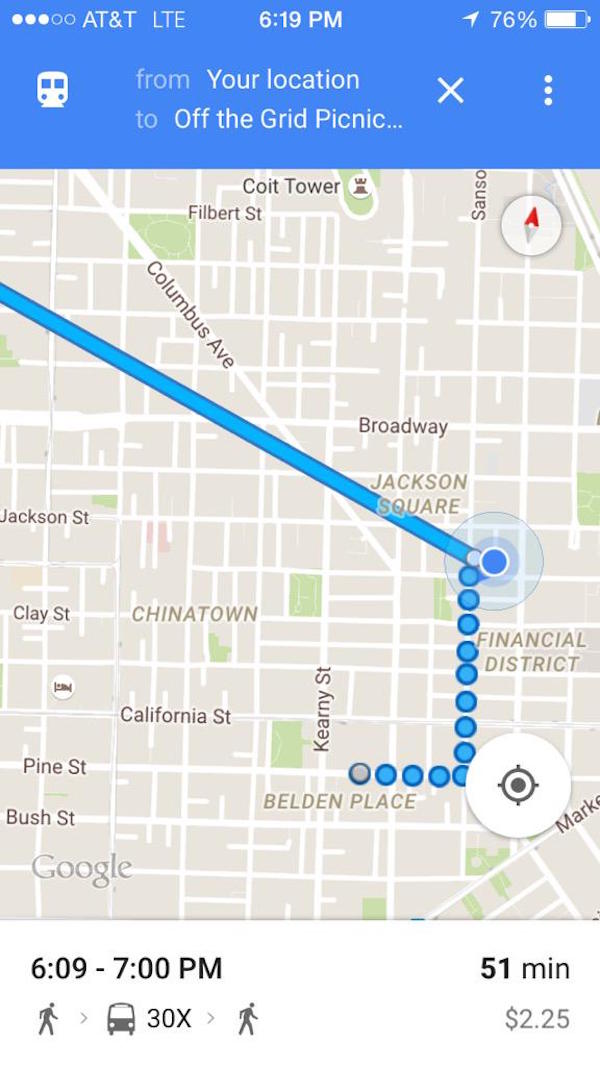This is a detailed caption for the provided image description:

"This image is a screenshot of Google Maps displayed on a smartphone. The map predominantly features gray and white shades, with key roads prominently highlighted. Columbus Avenue runs diagonally from the top left to the bottom right of the screen, while Broadway stretches horizontally from left to right. The Chinatown area is also visible within the map.

At the top of the screen, several status icons are displayed: the AT&T LTE signal indicator on the left, the current time "6:19 PM" in the center, and the battery level at 76% on the right. Beneath these icons is a blue banner, partially hidden, featuring a white bus symbol, and some text indicating a route from the user's location to a destination abbreviated as "off the grid picnic...". An 'X' icon is positioned to the right of this text.

The map itself is displayed below this banner, showcasing a standard map view without satellite imagery. A blue route line traverses the map from the upper left toward the lower right, passing Jackson Square, which is marked by a blue circle with a white border. Numerous small blue circles, akin to a string of pearls, indicate key points along the route. 

At the bottom of the screen, details about the trip are provided: a timeframe from "6:09 PM to 7:00 PM" on the left, the duration "51 minutes" on the right, and the cost "$2.25" listed beneath these details."